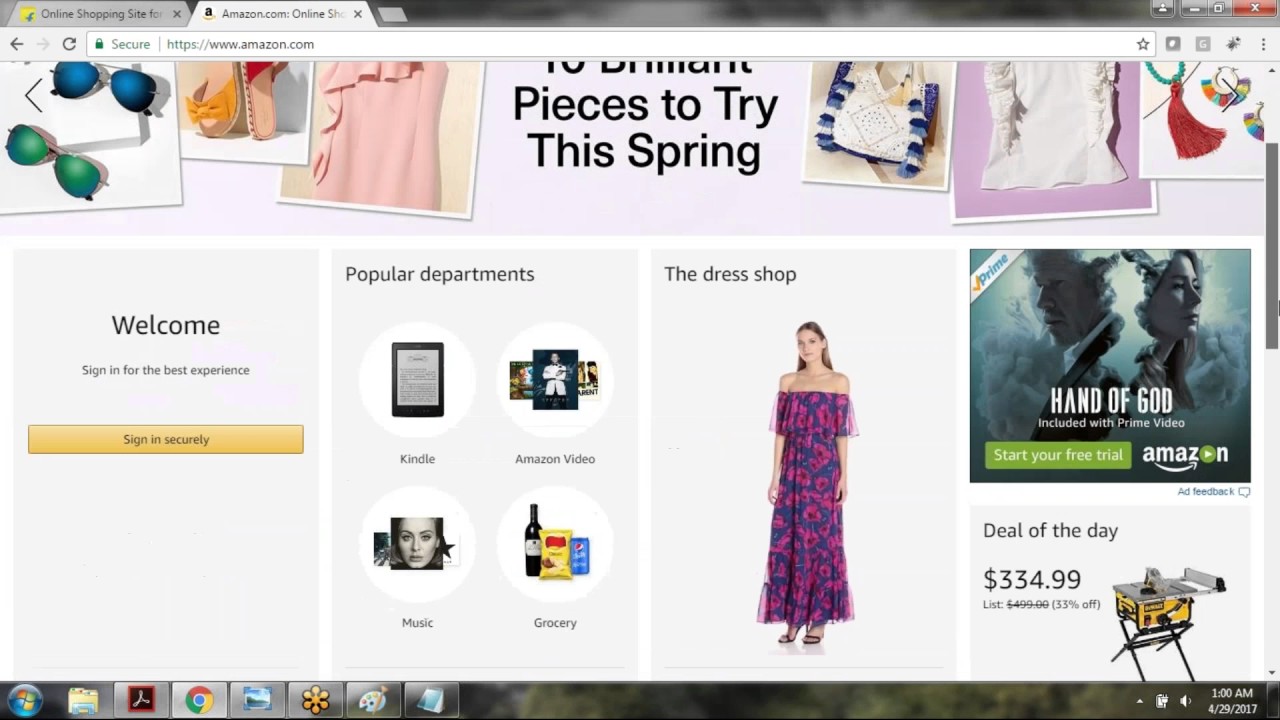The image displays a detailed view of a web browser window open to amazon.com. At the top are two tabs: the first is an online shopping site that can be closed with an 'X,' and the second is the currently active amazon.com tab, also closeable with an 'X.'

Below the tabs is the browser toolbar, including navigational buttons: a left arrow for 'back,' a right arrow for 'forward,' and a refresh icon in the middle. The address bar shows a secure URL: "https://www.amazon.com," and to the right of the address bar, there is a star icon for bookmarking and some additional icons for browser extensions or settings.

The main section of the webpage unfolds various elements of the Amazon homepage. On the upper left, there is a promotional banner featuring two pairs of sunglasses – one with green lenses and another with blue lenses – alongside a pair of sandals and a blouse. The banner header appears partially cut-off but hints at "10 pieces to try this spring."

Directly below this banner, various fashion items are displayed, including a handbag, a shirt, and pieces of jewelry such as earrings and a necklace.

Further down, there is a welcome prompt encouraging users to sign in securely for the best experience, along with a list of popular departments: Kindle, Amazon Video, Music, and Grocery.

Additional sections visible include "The Dress Shop," "Deal of the Day," and a mention of "The Hand of God," possibly referring to a featured product or promotion.